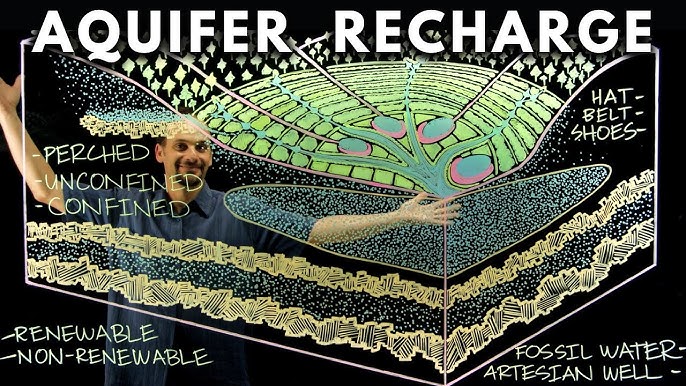The image is a detailed black and white poster titled "Aquifer Recharge," prominently displayed in bold white capital letters against a black background at the top. The upper portion of the poster features a green section depicting trees and leaves. The right side of the poster includes the words "Hats, Belts, and Shoes" at the top and "Fossil Water, Artisan Well" at the bottom. On the left side, the diagram illustrates different aspects of water interaction with the ground, including labels for "Perched, Unconfined, and Confined" in the center and "Renewable, Non-Renewable" at the bottom. At the heart of the image is a man with a tan complexion, possibly wearing a blue button-up shirt. He has dark hair, is balding, sports a mustache and a goatee, and appears to be presenting the information with one arm extended to the side and the other raised. The background shows an illustration of how water percolates through the ground into different aquifer layers, depicted by colored circles and a hand-drawn representation of the soil. The man is smiling, suggesting he is explaining or highlighting the importance of the processes shown in the poster.